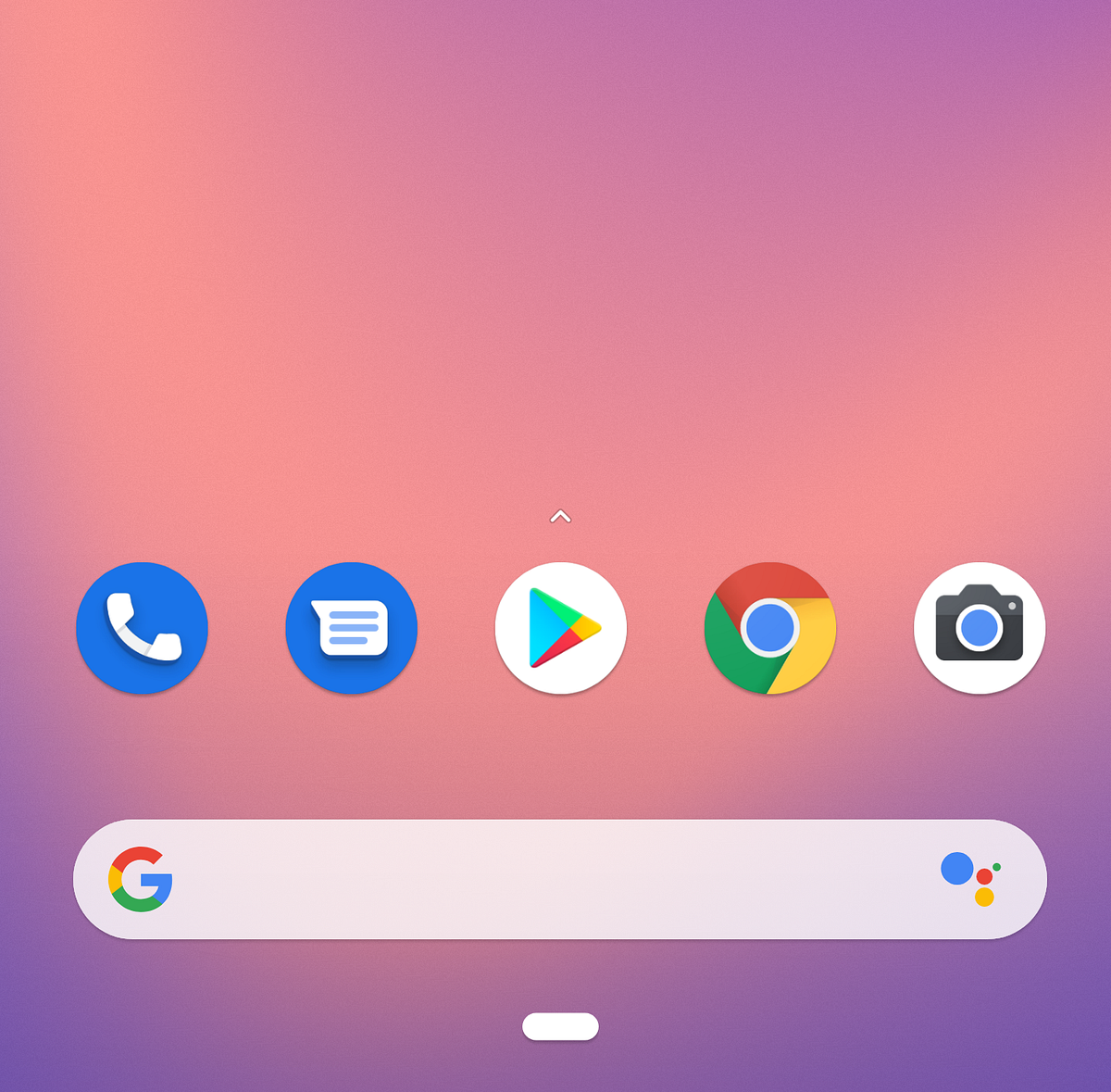The image is a screenshot of a phone screen with a striking gradient background that transitions seamlessly from medium purple to pastel salmon pink and periwinkle blue, creating an ombre effect. Superimposed on this vibrant backdrop are five prominent circular buttons arranged in a horizontal lineup. 

1. The first button is a vivid blue circle featuring a white phone symbol at its center.
2. The second button, also in bright blue, displays a white chat bubble icon.
3. The third button is a white circle containing the Google Play Store logo, represented by a multi-colored play button in shades of green, blue, orange, and pink.
4. The fourth button showcases the Google Chrome logo - a blue circle in the center, outlined in white, with segments in red, yellow, and green forming the outer circle.
5. The fifth and final button is a white circle with a black camera icon. The camera icon includes a blue lens outlined in white and a small gray button in the upper right corner.

Below these buttons is a Google search bar. This bar is light gray and spans the width of the phone screen, featuring rounded edges. In the far left corner of the search bar is Google's multicolored "G" logo in red, yellow, green, and blue. The far right side features a series of multicolored dots in varying sizes—a large blue dot, a small green dot, a medium-sized yellow dot, and a medium-sized red dot. Positioned beneath the primary search bar is a smaller, similarly shaped light gray box, which appears stubby in comparison.